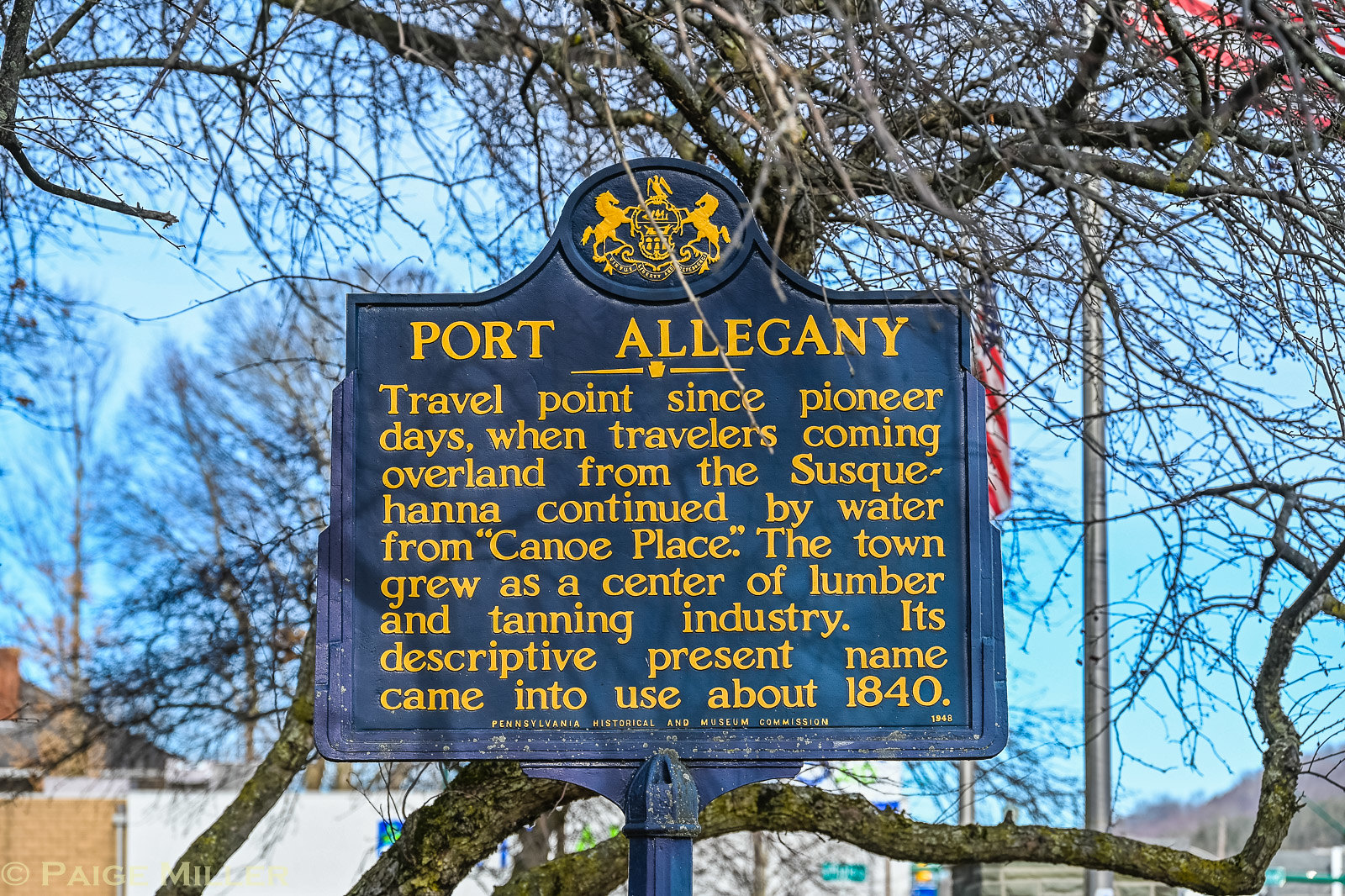This outdoor photograph features a dark blue metal historical sign, prominently positioned at the center of the image. The sign is detailed in bright yellow lettering, which contrasts vividly against the dark blue background. At the top of the sign is an ornate crest, depicting two horses facing each other, flanking a banner with flags and an eagle. Below the crest, the sign reads: "Port Allegany - Travel point since pioneer days when travelers coming overland from the Susquehanna continued by water from the Canoe Place. The town grew as a center of the lumber and tanning industry. Its descriptive present name came into use about 1840." 

In the backdrop, leafless tree branches suggest a winter setting, with a partial view of an American flag flying against a clear blue sky. A few buildings can be seen in the distance, providing context to the sign's historical narrative. Additionally, a translucent copyright mark is visible in the lower left, reading "Page," partially obscured by the photo's background elements.